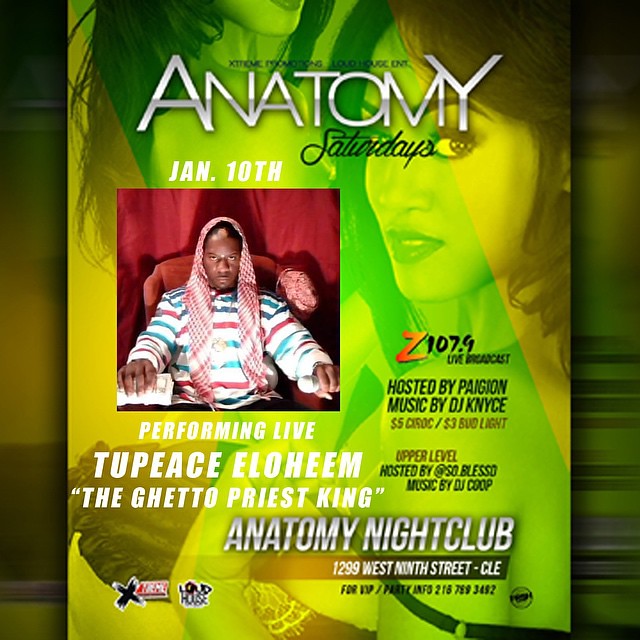This vibrant poster, predominantly featuring shades of yellow and different greens, advertises an event at Anatomy Nightclub, located at 1299 West 9th Street. The title "Anatomy Saturdays" is prominently displayed at the top in white and black letters. The poster centers around a square photograph of a man sitting on a sofa, indicating that he will be "Performing Live: Peace Elohim, The Ghetto Priest King." 

To the right of this image, the radio station sponsor Z107.9, with the Z in orange, is highlighted, along with the information that the event is hosted by Pagione and features music by DJ Gneiss. Additional details include promotions such as "$5 crock, $3 quad light." 

Beneath this section, the upper level details specify that it is hosted by So Blessed with music by DJ Coop. The bottom section of the poster reinforces the location, Anatomy Nightclub, and includes the promoter's name, Xtreme, and the Loud House symbol.

The background is artistically adorned with a drawing of two women with dark hair and low-cut dresses, who appear to be looking directly at the viewer, enhancing the poster's visual appeal. The date of the event, January 10th, is also mentioned, ensuring attendees have all critical information.